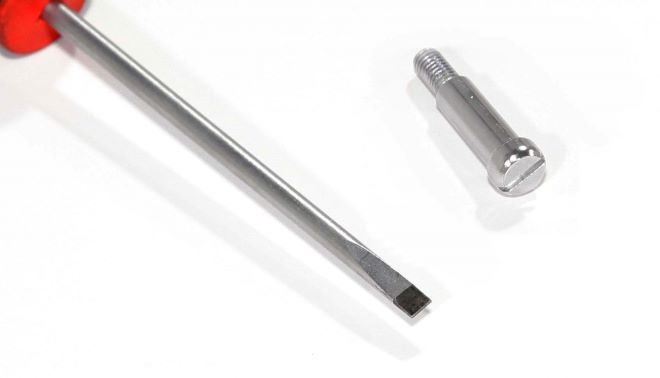The photograph features a close-up view of a flathead screwdriver and a screw on a white tabletop. The handle of the screwdriver, partially visible in the upper left corner, is red and round, leading to a long metal shaft approximately 5 to 6 inches in length. The shaft terminates in a black, magnetized flathead tip. To the right of the screwdriver, there's a large silver screw, identifiable as a straight-edge screw. The screw has a partially threaded shaft with the threads extending up from the pointed end about a quarter to a third of the way towards the smooth, cylindrical section that leads to the screw head. Both the screwdriver and the screw cast shadows on the white surface, with reflections of light highlighting their metallic finishes.